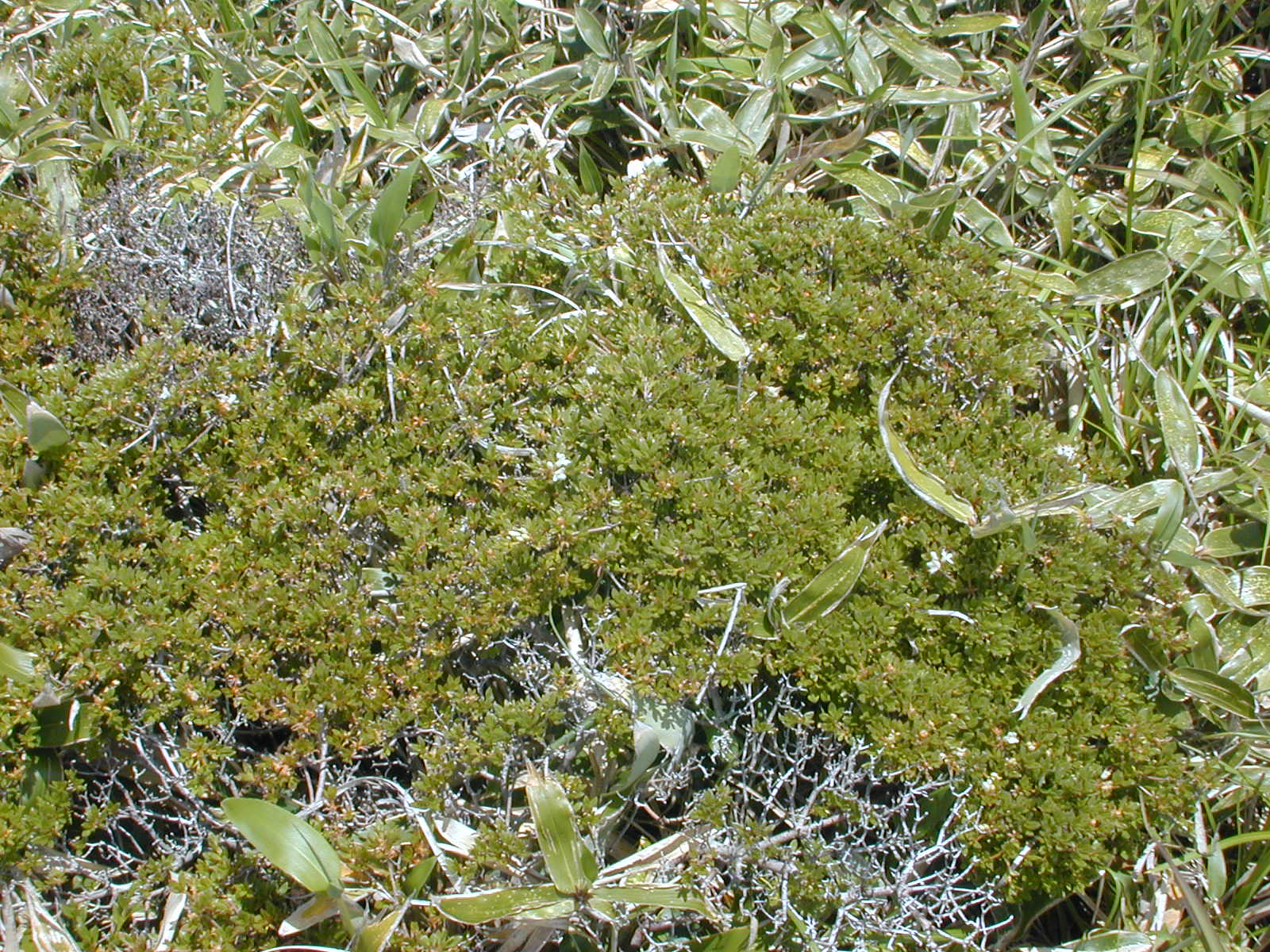This captivating outdoor photograph showcases a richly textured piece of land, brimming with various shades of green and a diversity of plant life. At the very bottom, there are a few slender, glossy plants with about three leaves each, accompanied by small, almost white twigs that resemble bare, leafless bushes. Above this sparse layer, the scene transforms into a dense conglomerate of smaller, clover-like plants, creating a deep green patch at the center. Scattered throughout the area are longer leaves with a glossy, lighter green hue, interspersed with white, silvery twigs which might even host some thorns. Taller grass stems weave through the foliage, adding to the wild, overgrown quality of the landscape. On the right-hand side, some plants appear to have been flattened or broken, suggesting the area has been disrupted. The overall effect is a vivid, untamed swath of greenery, revealing a harmonious mix of moss, grass, and various clusters of leaves and foliage.